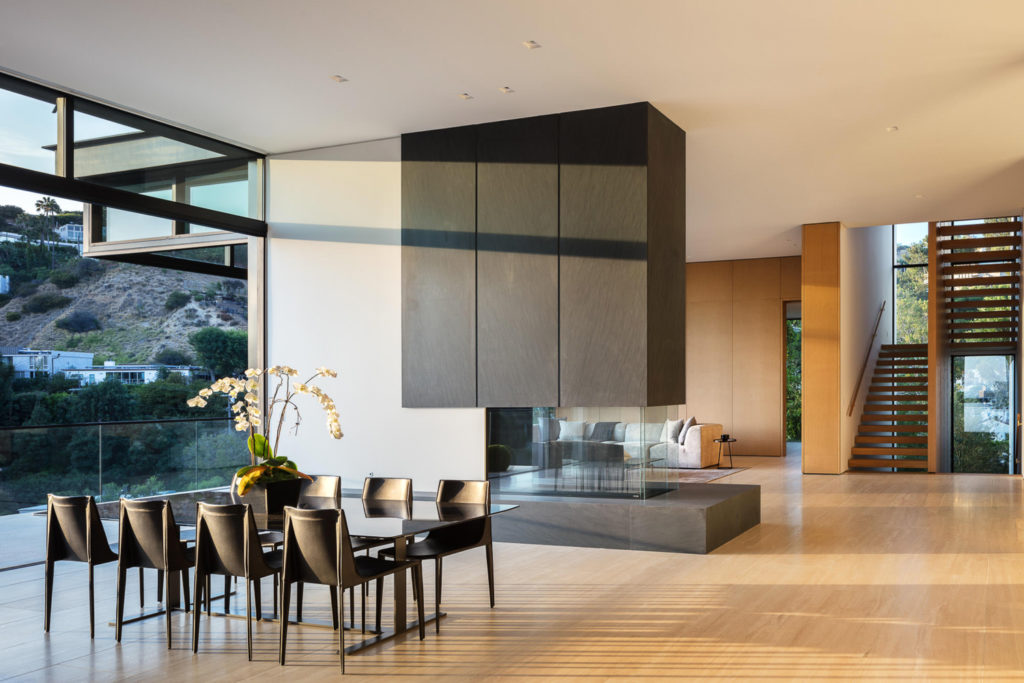This professionally photographed image showcases a spacious and modern open-concept home, emphasizing a harmonious blend of various design elements. Dominating the center of the room is a sleek rectangular glass dining table accompanied by eight black chairs neatly tucked under it, four on each side. A stylish vase with yellow and green leaves and white flowers sits atop the table, adding a touch of freshness and elegance. 

To the left, an expansive wall of windows offers a breathtaking view of a hillside, dotted with green trees, gray rocks, and even some white buildings, hinting at a possible Californian setting, perhaps near the Hollywood Hills. The sunlight streams in, illuminating the light brown hardwood floors that extend throughout the area. 

A stark white, structural wall with a distinctive black cube art piece featuring three vertical rectangles serves as a modern focal point. Adjacent to the dining area is a living space with a beige couch and solid light brown walls that match the flooring, creating a warm and cohesive aesthetic. 

In the background, a set of wooden stairs with zigzag steps ascends to a landing before continuing upward, presumably to the second level of the home. Brown cabinets, reminiscent of large blocks, offer storage while maintaining the room’s modernist appeal. The overall atmosphere of the room is one of sophisticated elegance, perfectly captured in this high-quality, magazine-worthy photograph.